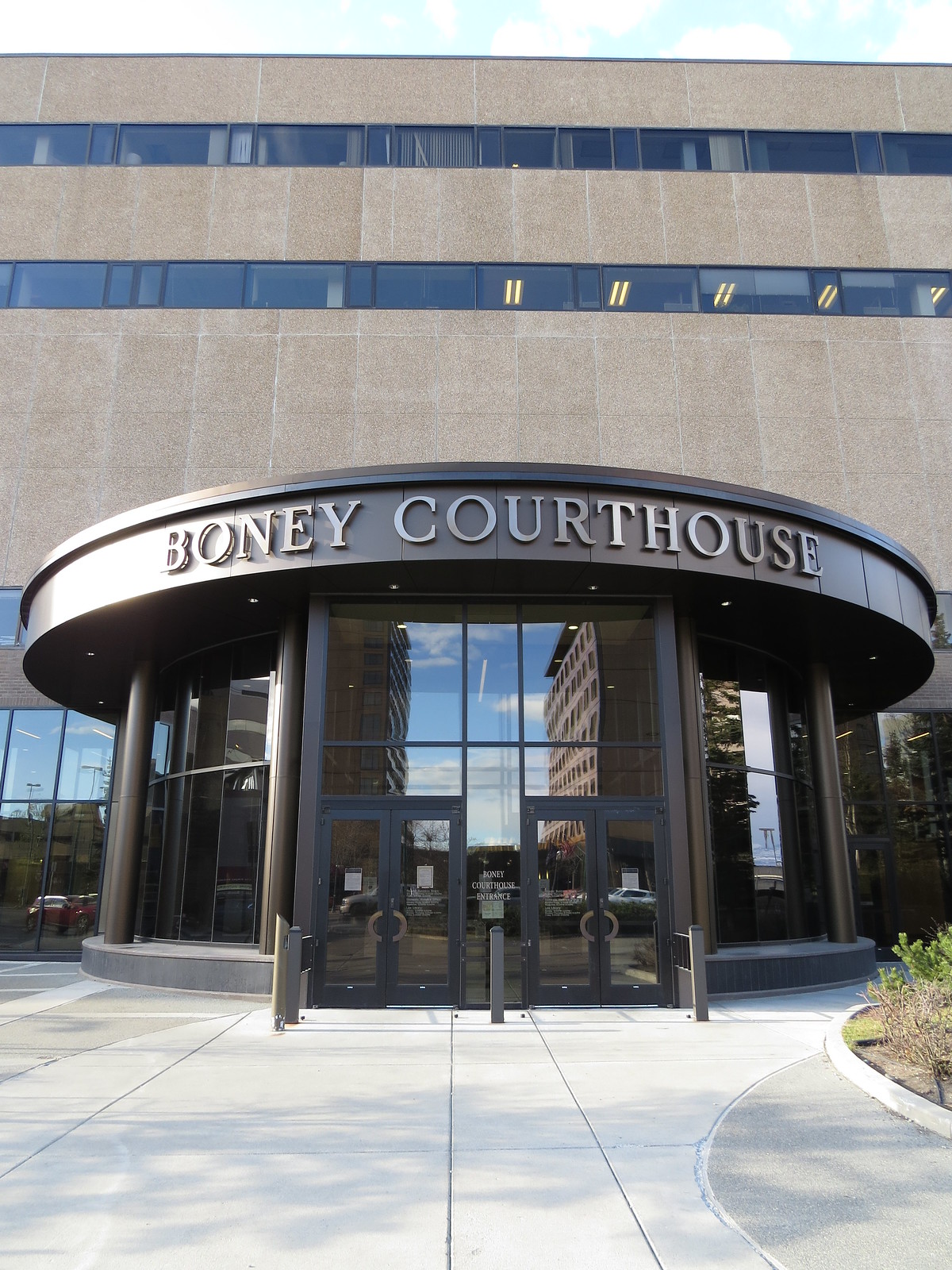The image depicts the entrance of the Boney Courthouse, a prominent building characterized by its light brown and gray concrete façade. The name "Boney Courthouse" is clearly displayed in large, capital letters across the top of the entrance. The entrance itself features four clear double doors with black frames and brownish knobs, flanked by multiple windows. Reflections in the doors and windows reveal surrounding buildings, blue skies, clouds, and cars. The front area includes a clean gray concrete walkway, several posts, and a median with plants. The building stands approximately five to seven stories high, with windows adorned with black horizontal streaks and visible interior lights. To the right of the image, there is additional greenery, including grass and shrubs. The courthouse's design includes a circular entrance section with substantial glass paneling, adding to its modern appearance.